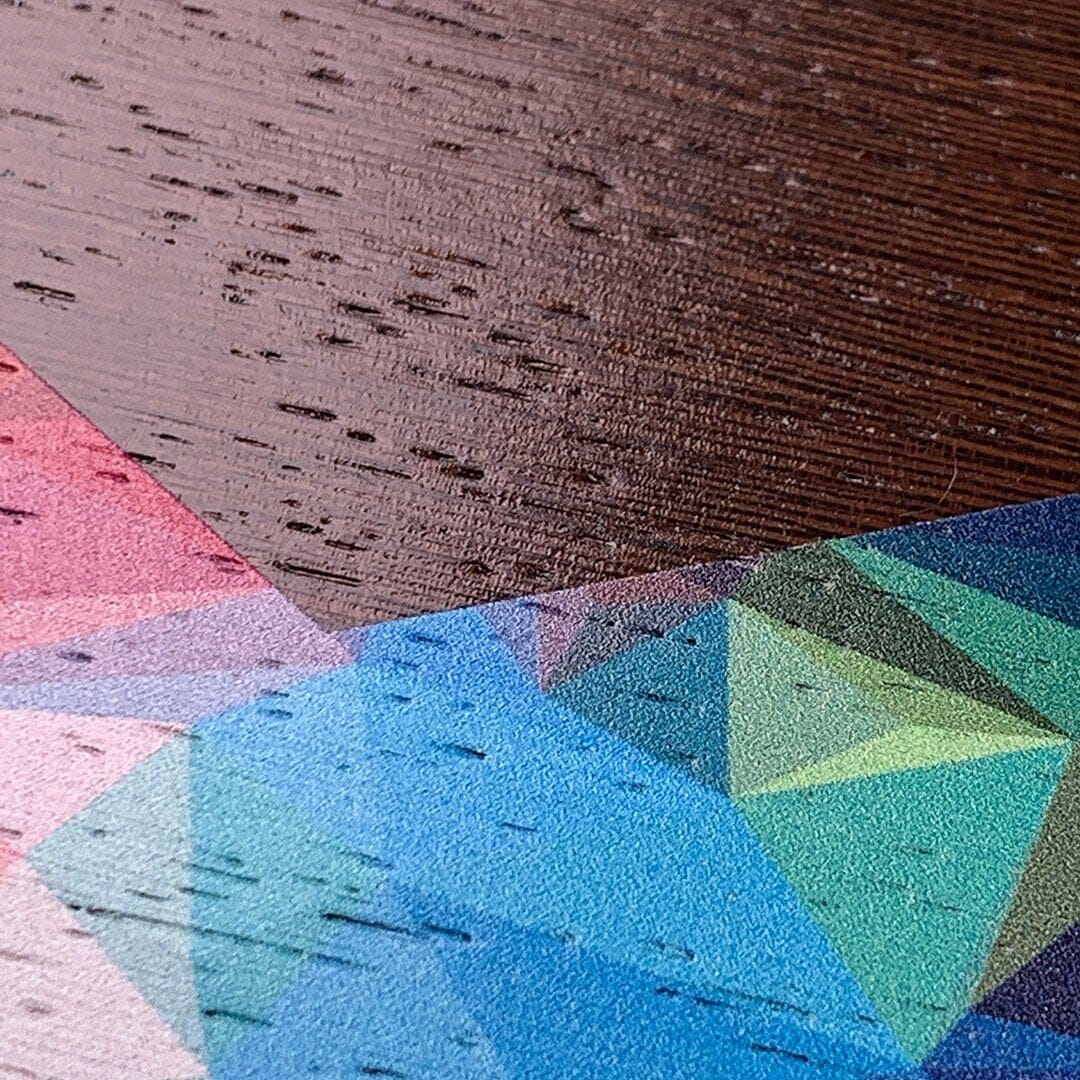This close-up image features a piece of wood, the top half of which is painted in a chocolate brown or reddish-brown color. The natural texture and grain of the wood are visible, along with numerous indentations and pit marks which suggest it has been either pounded or rolled over. The bottom half of the wood is a vivid array of multicolored, angular, semi-transparent geometric shapes - including triangles and trapezoids - that create a kaleidoscopic effect. A V-shaped line separates the brown upper section from the colorful lower part. On the left, shades of pink and red dominate, transitioning into blues and teals in the middle, and finally into yellows, greens, and earthy browns on the right. The underlying texture of the wood is still discernible through the multicolored paint, emphasizing the imperfections beneath.